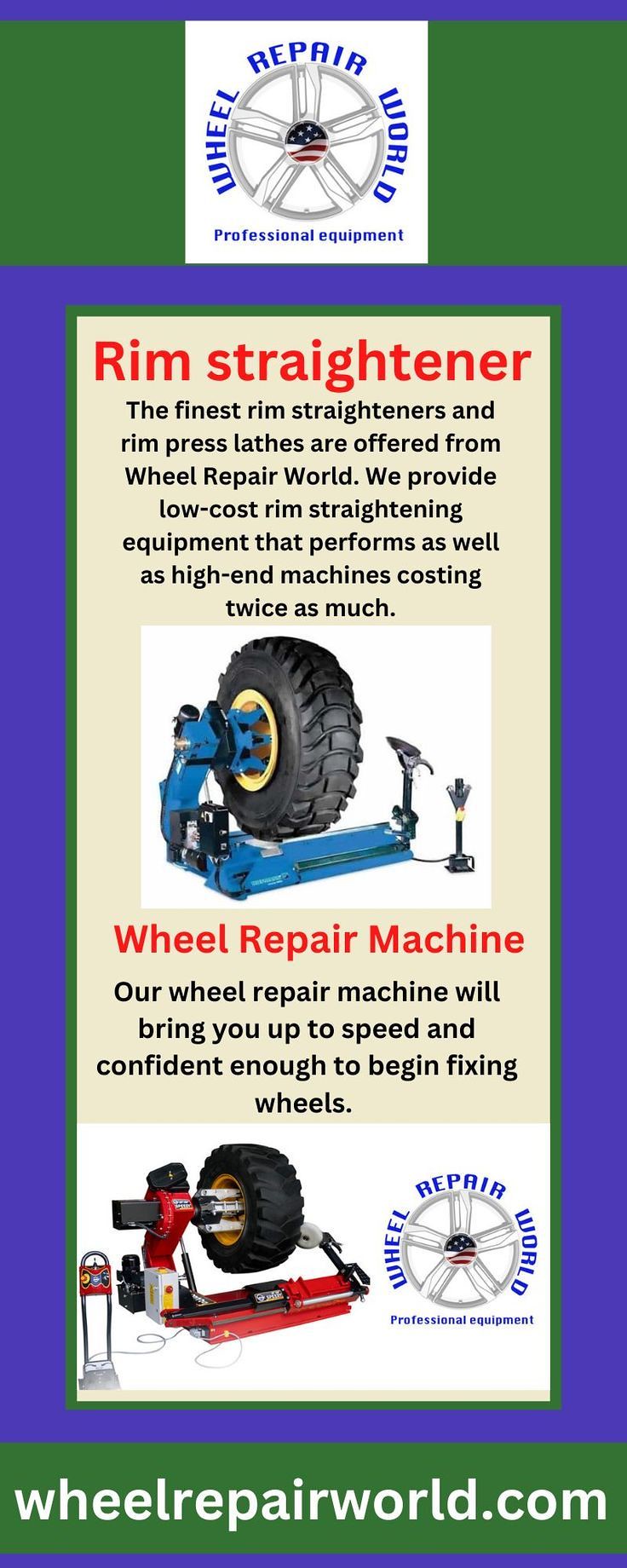The image is an advertising poster for Wheel Repair World, showcasing their professional equipment for tire repairs. At the top, the logo "Wheel Repair World" is prominently displayed within a circular design, surrounding an image of a wheel with spokes and an American flag in the middle. This is followed by the focus on two primary products: the Rim Straightener and the Wheel Repair Machine. 

The first section elaborates on the Rim Straightener, with the text: "The finest rim straighteners and rim press lathes are offered from Wheel Repair World. We provide low-cost rim straightening equipment that performs as well as high-end machines costing twice as much." Accompanying this is an image of the rim straightener, which appears to be blue in color.

Beneath this, the ad highlights the Wheel Repair Machine, with the text: "Our Wheel Repair Machine will bring you up to speed and confident enough to begin fixing wheels." There is a corresponding image of the wheel repair machine, which seems to be red and similar in structure to the rim straightener, featuring a base with a raised mechanical arm designed to hold and spin wheels for repair.

On the side, the phrase "Wheel Repair World Professional Equipment" is reiterated, emphasizing the quality and professionalism of their offerings. At the bottom of the poster, the website "wheelrepairworld.com" is displayed.